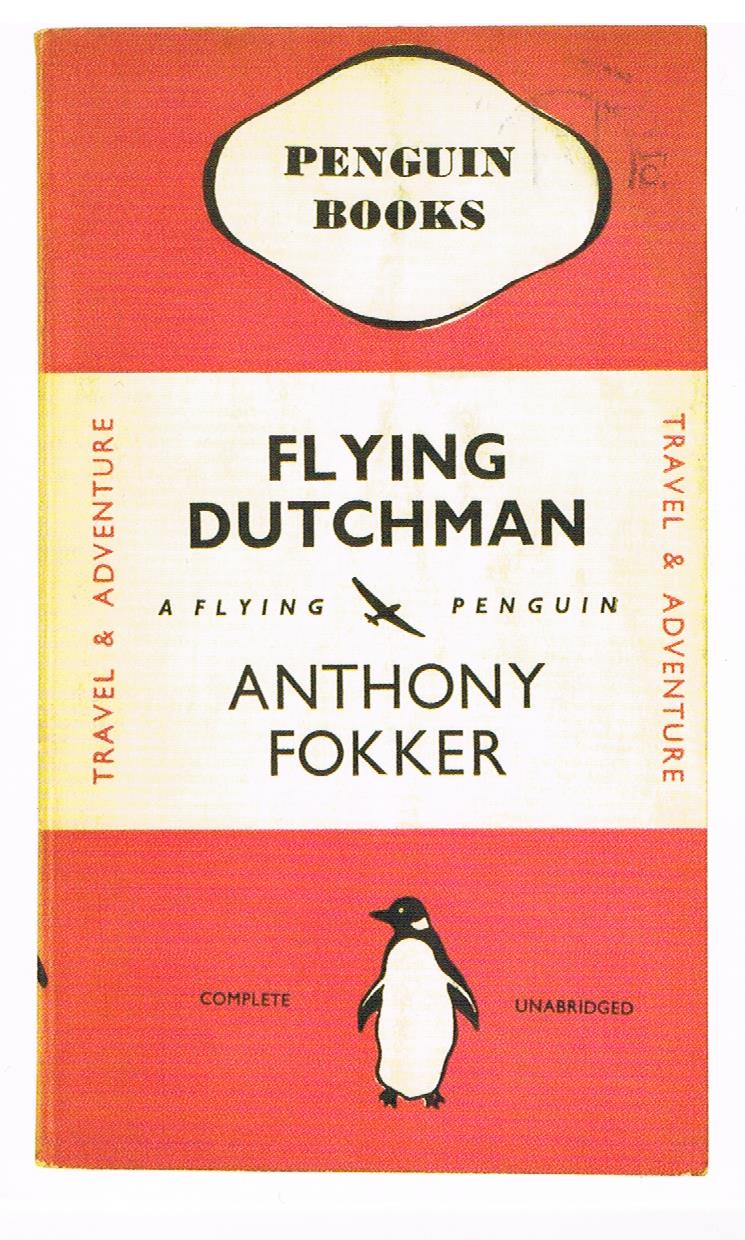This image is of the cover of an older, pocket paperback book titled "The Flying Dutchman" by Anthony Fokker. The cover features a classic Penguin Books design, with an orange panel at the top and bottom, sandwiching a white banner across the middle. The top orange panel contains the Penguin Books logo in a white bubble with a black border, and the text is capitalized in black. The middle white section holds the book's title, "The Flying Dutchman," which is aligned sideways, and also includes the subtitle "A Flying Penguin." In this section, there are small illustrations, including an airplane, and above and below the title, the text "Travel and Adventure" appears. The author's name, Anthony Fokker, is prominently displayed in black font. The bottom orange panel features another illustration of a walking penguin with its arms outstretched, and next to it the words "Complete Unabridged." Despite its age and a bit of visible dirt, the cover's iconic design and layout distinctly mark it as a Penguin Books travel and adventure series publication.